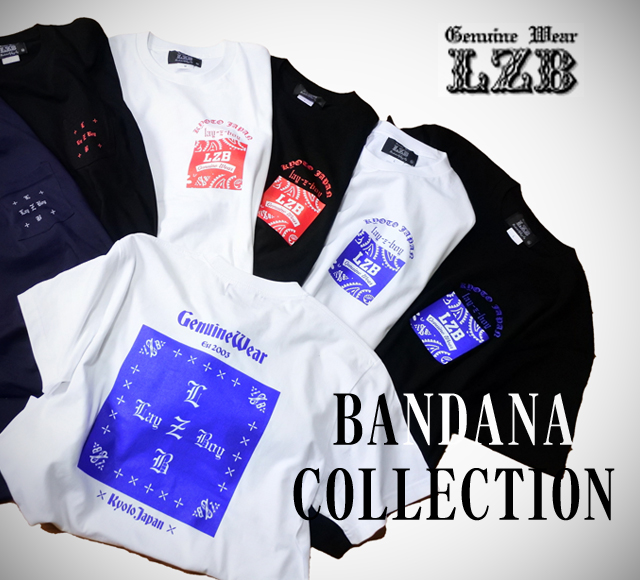The image is a top-down view of an advertisement showcasing a collection of seven t-shirts. The background is predominantly white with gradient effects, creating a clean and modern look. Six of the t-shirts are fanned out in a semi-circle, with the colors arranged from left to right as blue, black, white, black, white, and black again. A seventh white t-shirt lies prominently on top of these. Each t-shirt features distinct graphical designs with logos in either blue or red. The t-shirt on top has a detailed logo that reads "Genuine Wear, Established 2003, Lazy Boy, Kyoto, Japan". In the top right corner of the image, text reads "Genuine Wear LZB" in an elegant font, highlighting the brand. In the bottom right corner, the text "Bandana Collection" appears, some letters in black and some turning to white as they overlay a black t-shirt beneath, giving a dynamic visual effect. Overall, the image serves as a sophisticated promotional advertisement for LZB's Bandana Collection of t-shirts.